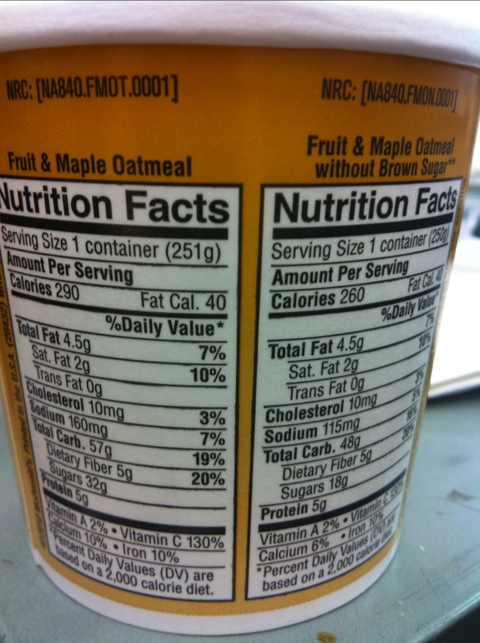This photograph captures a close-up view of a cylindrical paper carton of oatmeal, prominently labeled as "Fruit and Maple Oatmeal without Brown Sugar." The container is primarily orange, transitioning to white near the base, and features black text against this background. The top of the lid is white. Black text on the container includes details such as "NRC" and the identification number "NA84.FM0T.0001." The nutritional facts panel is displayed in white with black text, bordered by a smaller black rectangle. Key nutritional information is meticulously detailed: the serving size is one container, containing 260-290 calories, 4.5 grams of total fat, 2 grams of saturated fat, no trans fat, 10 milligrams of cholesterol, 115-160 milligrams of sodium, 48 grams of total carbohydrates, 5 grams of dietary fiber, 18 grams of sugar, and 5 grams of protein. The container is situated on a light blue table, with a white ledge visible on the right side, suggesting the photo was taken outdoors.